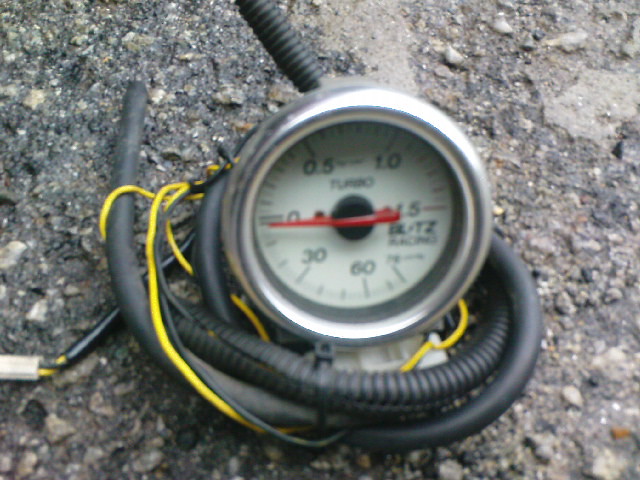This image showcases a detached speedometer-like dial set against a rough, broken concrete surface embedded with small rocks. The dial, covered by glass, features a red needle currently pointing to the 0 mark, positioned at the west side of the dial. The face of the dial is white, adorned with long black slash marks corresponding to numbers and shorter, unnumbered slash marks in between. Key numerical graduations include 0.5 at the upper left, 1.0, 1.5 at the east, 6.0 near the south, and 30 before returning to 0.

Below and to the side of the dial, a bundle of yellow and black wires is visible, curled and slightly disordered. One black plastic wire casing, noticeable for its ridges, is cracked along its length, exposing the wires within. The detached nature and the detailed state of the wires and dial suggest that this instrument was once an integral part of a mechanical system, now rendered inoperative and abandoned on a jagged concrete expanse.